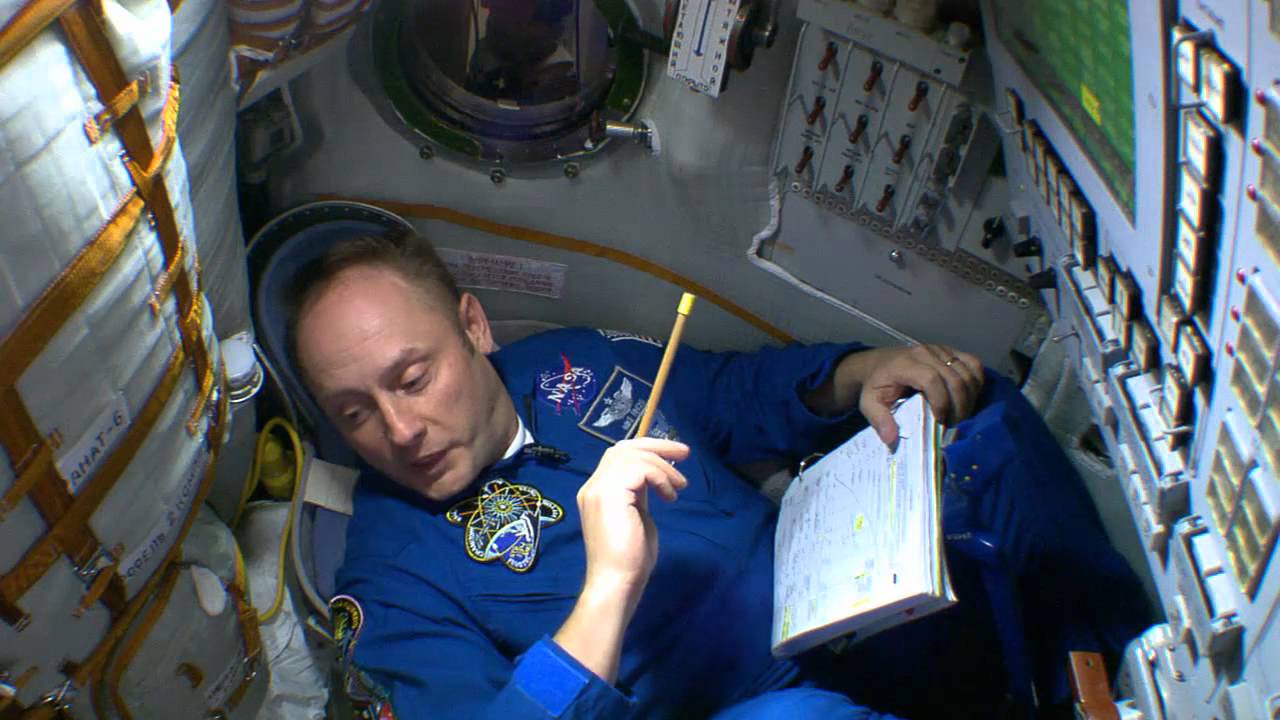This photograph captures a middle-aged, balding male astronaut, likely aboard the International Space Station or a similar spacecraft. The astronaut is dressed in a blue coverall uniform adorned with a NASA logo on his left shoulder and an illegible logo on his right shoulder. He mirrors the appearance of Elon Musk with his thinning hair and thin lips. Positioned in a very tight, cramped capsule, he lies in a semi-reclined position with his knees propped up. The astronaut holds a yellow pencil in his right hand while his left hand secures an open white ring-bound notebook on his knee. He appears to be meticulously recording data or calculations based on readings from various electronic components and control panels lining the capsule walls. The background is predominantly white, featuring a blend of buttons, switches, and computerized screens. Notably, a green screen and a small porthole interrupt the sea of white, black, and gold-colored controls. The astronaut's attention is directed off to his right, possibly engaging in a data collection process or conversing with someone off-frame. His surroundings, including puffy materials with orange stripes and a control unit, emphasize the confined and functional environment essential for space missions.